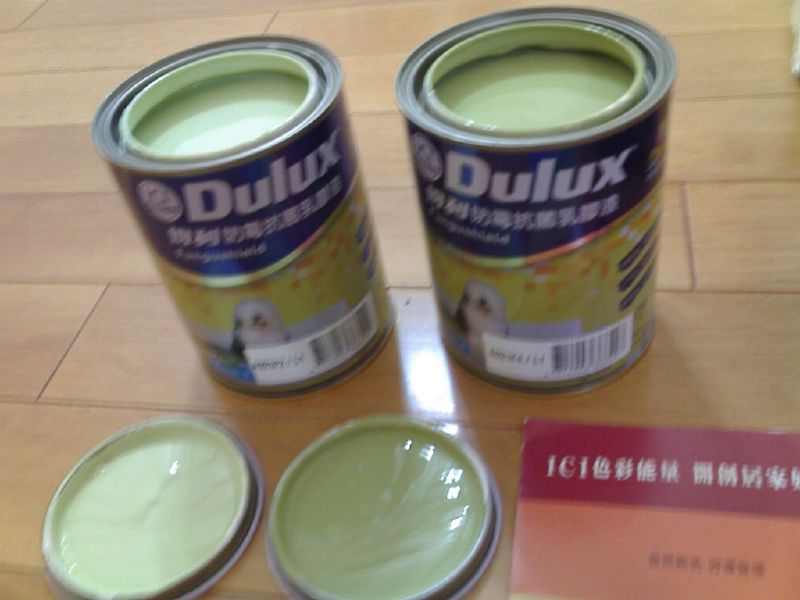The image is a slightly out-of-focus color photograph in landscape orientation, depicting two identical metal paint cans with their lids removed and lying in front. The brand name "Dulux," spelled D-U-L-U-X, is prominently displayed in white letters on a dark blue background on each can. Beneath the brand name, there are some writings in Asian characters. Each can also features an image of a wall-painted background with a white and green bird or a sheepdog, which has yellow accents beneath its eyes or is situated in front of a yellow background. Furthermore, there is a UPC barcode on the lower part of each can. The paint in both cans is a pale mint green color, although the left can's contents seem slightly lighter in shade. The metallic lids, placed in the foreground, also display this mint green paint on their undersides. The bottom right corner of the photograph shows a cut-off, rectangular, red and orange brochure with white Asian typography and the letters "ICI" visible. The beige-gray floor beneath appears to be golden honey oak plank flooring, adding a warm contrast to the cool tones of the paint and the metallic sheen of the cans.